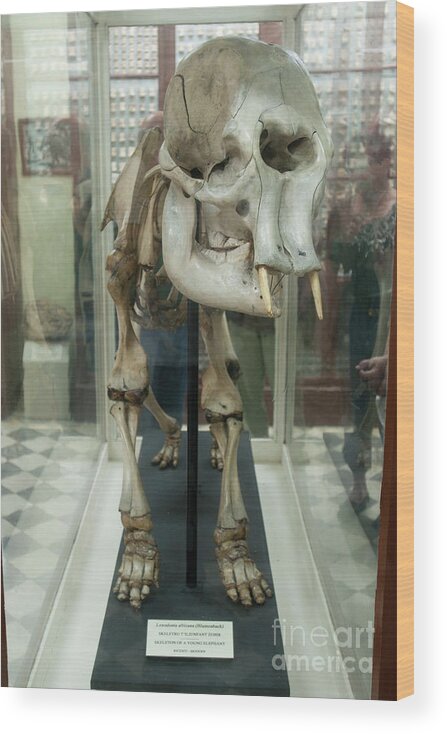The image is a rectangular, six-inch-high by three-inch-wide photograph displayed on a canvas with light brown edging on the right side, giving the impression that the right side is closer to the viewer. The photograph, taken indoors at a museum, captures a fossilized four-legged creature encased in a plexiglass enclosure. The fossil showcases a large bulbous skull with a strong lower jaw, featuring two very small, short tusks or horns protruding near the top of the jaw, along with wide eye sockets and a large central nasal cavity. The skeleton is supported by a black rod connected to the floor. A small, white rectangular plaque sits just above the rod support beam, though its text is unreadable due to blurring. In the background, the blurred image of another visitor can be seen examining the display. In the lower right-hand corner of the photograph, "Fine Art America" is printed in light gray text.